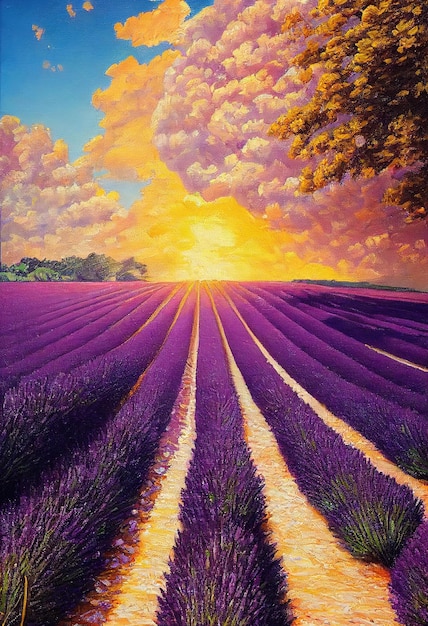The image is a captivating digital painting in portrait mode, depicting an expansive lavender field under a vibrant sky. The lavender plants stretch vertically toward the horizon in the middle of the image, creating a mesmerizing sea of bright purple hues. Among the lavender, golden stripes run down the center of the fields, adding a striking contrast to the scene. Above the horizon, a line of distant trees frames the landscape. The sky above is a brilliant, rich blue, with a setting sun casting golden light on the clouds. The clouds themselves are a stunning mix of dark yellow to light yellow at the center, blossoming out into purplish tones that mirror the lavender fields below. In the top right-hand corner, there's a tree with light brown leaves, set against a backdrop of puffy clouds in shades of light pink, dark pink, and orange. The intricate, oil paint style and the vivid colors make the lavender look especially beautiful against the dramatic, colorful sky.